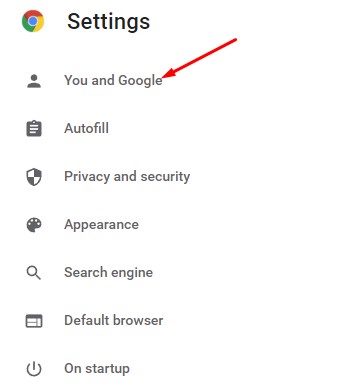This detailed caption describes a screenshot of a side menu, likely from Google or Google Chrome:

---

The image is a screenshot of a Google side menu, featuring a series of headers accompanied by icons. At the top left, the recognizable Google insignia is displayed. This insignia consists of a circle segmented into three colors: red on top, yellow on the right, and green on the left, with a smaller blue circle in the center. Below the insignia, the text "Settings" is written in black against a white background, with all menu items featuring black lettering on the same white background.

The side menu includes the following items:

1. **You and Google:** Indicated by an icon depicting a person, this header has a long red arrow pointing to it, suggesting that the user is currently in this section or it is being highlighted for attention.
2. **Autofill:** Represented by an icon of a piece of paper with lines on it.
3. **Privacy and Security:** Displayed with a shield icon.
4. **Appearance:** Marked with a palette icon featuring dots to symbolize various colors for painting.
5. **Search Engine:** Accompanied by a magnifying glass icon.
6. **Default Browser:** Identified by an icon of a computer screen.
7. **On Startup:** Shown at the bottom with an icon resembling a power button.

This menu visually guides the user through various settings and customization options within Google or Google Chrome.